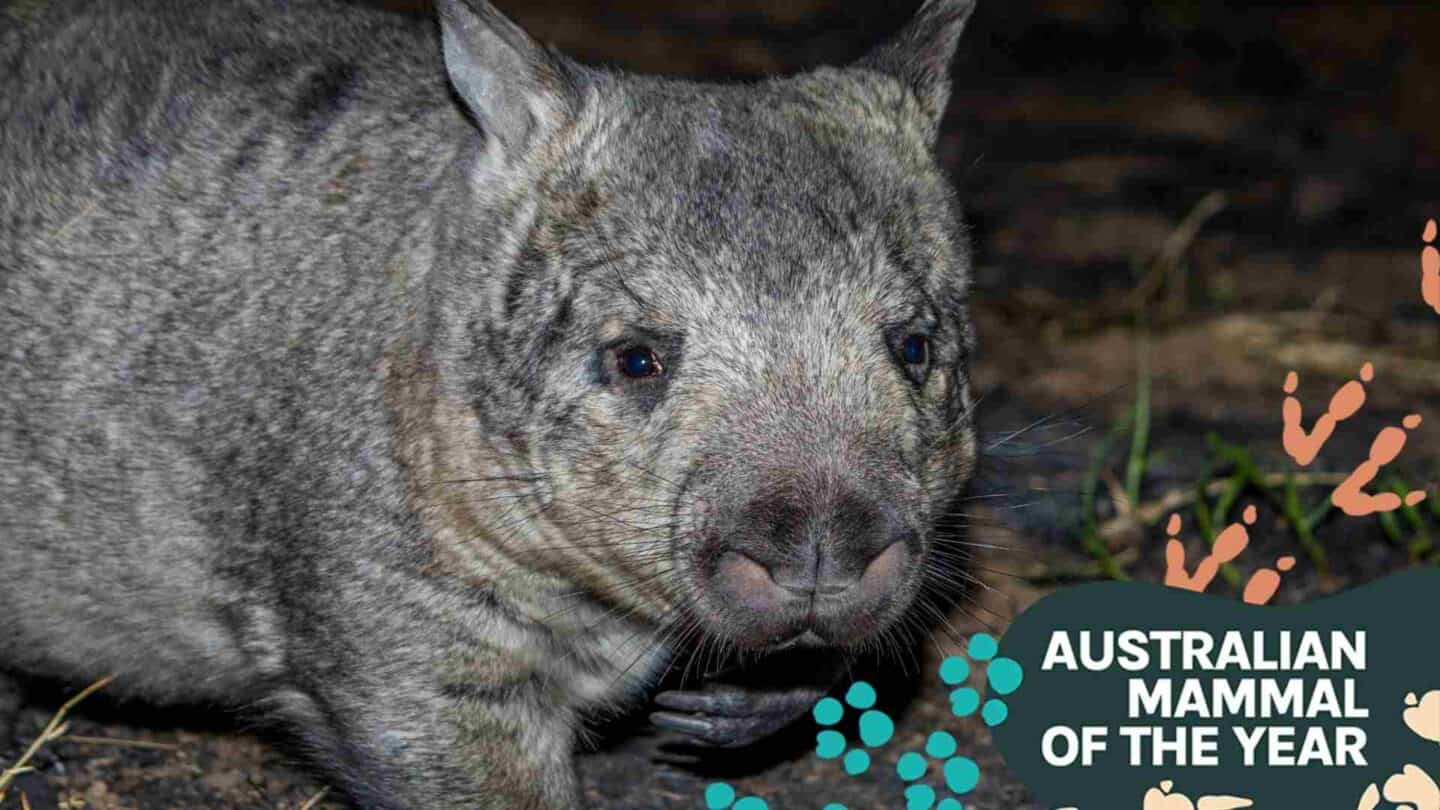In this image, we see the Australian Mammal of the Year, announced in bold white text set against a dark background. The text, “Australian Mammal of the Year,” is prominently displayed, either enclosed in a dark blue squiggly circle or in simple white capital letters standing out clearly. The setting is nighttime, with only a few visible strands of grass emerging from the ground, giving it a dim, mysterious ambiance.

The focal point is a large, gray, furry animal that resembles a wombat, standing about three feet tall with round, black beady eyes, perky ears, and a distinctive pig-like snout. The animal is facing towards the right but looking directly at the camera, with its left paw raised toward its mouth, giving it a somewhat innocent and curious expression. The lighting predominantly illuminates its face, making its features stand out against the darkened backdrop.

Enhancing the scene, various stylized paw prints are scattered across the image. A group of four turquoise blue paw prints is visible, with additional tan paw prints located in the bottom right corner. On the left side, possibly diagonally across or going up the side of the page, there are pinkish-salmon-colored jointed paw prints, adding a whimsical element to the composition. The footprints range from bird-like to other unidentified animal prints, colorfully decorating the scene and providing additional texture and interest to the image.